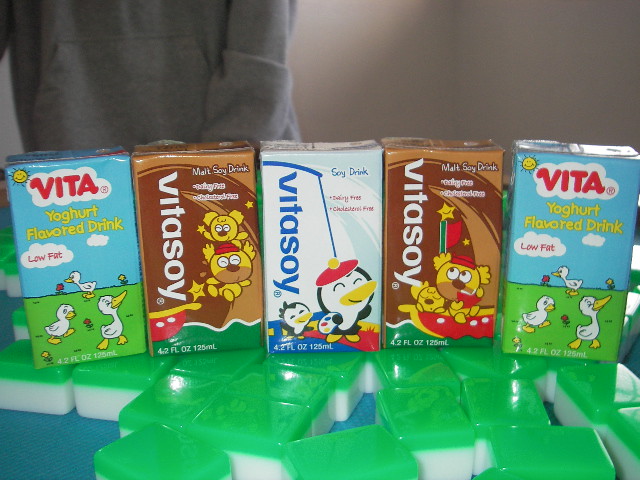This photograph showcases an assortment of dairy and soy-based beverages displayed in five distinct containers. On the far left and far right, you will find containers labeled as Vita Yogurt Flavored Drink, each adorned with charming cartoon ducks against a vibrant backdrop. Adjacent to these containers are brown-packaged Vita Soy drinks, each featuring an endearing bear illustration. Centrally positioned is another Vita Soy container, distinctively decorated with two playful penguins. All five containers are placed atop green-and-white rectangular storage boxes with lids. In the background, a person wearing a gray sweater can be seen, adding a subtle human element to the scene.